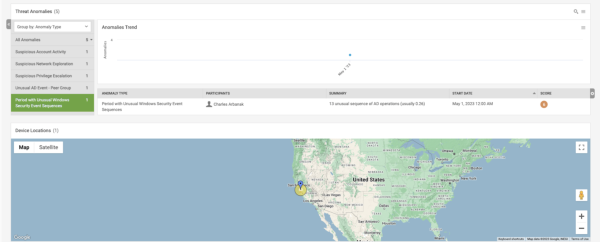The image is a detailed screenshot of a digital map interface, prominently displaying the United States surrounded by oceans. At the center, a yellow pin is dropped on California, indicating a specific point of interest. The top of the image features a search bar, accompanied by several menu options aligned along the left side. On the right side, there is a text box that contains a customer's shipping information, including a summary and a start date listed as May 1st, 2022, at 12:00 AM. The map interface includes buttons for zooming in and out, enhancing the utility and navigability of the map. This appears to be a scheduling or tracking platform, likely used for managing logistics or deliveries.